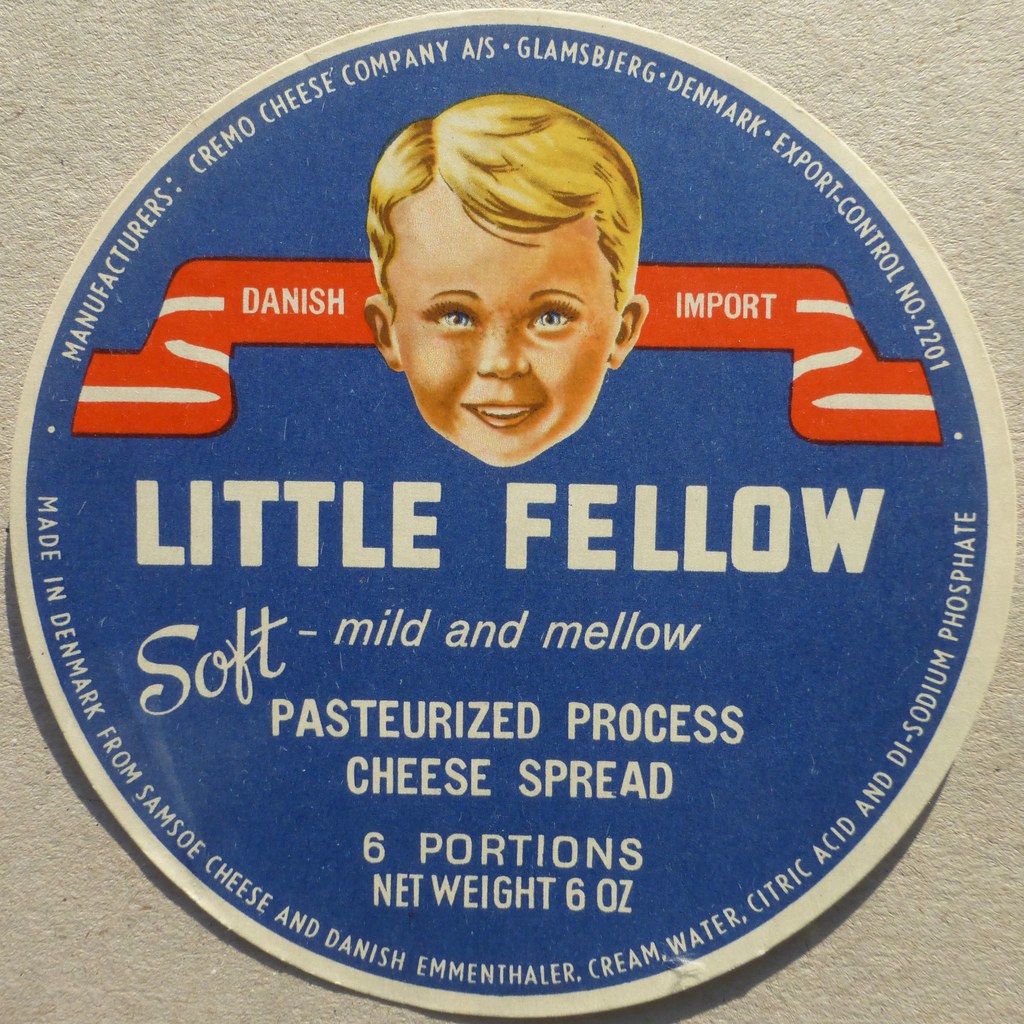This is a detailed label for "Little Fellow Soft Mild and Mellow Pasteurized Processed Cheese Spread" weighing six ounces, divided into six portions. The container is round and has a blue background. At its top center, a red ribbon design features a little boy with blonde hair and blue eyes, and the words "Danish Import" in white letters. Surrounding the circle in white font, it reads "Manufacturers, Cremo Cheese Company, AS Glamsberg, Denmark, Export Control Number 2201." Beneath the boy's face, the brand name "LITTLE FELLOW" is displayed in all caps, with "SOFT" written in cursive, followed by "MILD and MELLOW" and "PASTEURISED PROCESSED CHEESE SPREAD" underneath. Further details include "SIX PORTIONS" and "NET WEIGHT, 6 ounces." Along the bottom half of the circle, it lists the ingredients: "Made in Denmark from Samso Cheese and Danish Emmerthal cream, water, citric acid, and disodium phosphate."